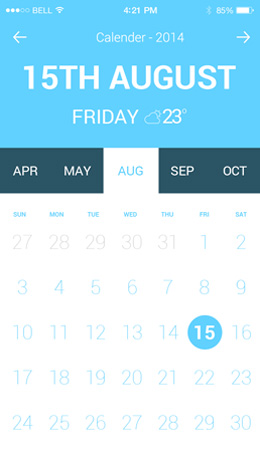This image is a cropped screenshot of a mobile calendar interface, which appears stretched, wide, and enlarged. At the top, the header is rendered in light blue. Centered at the top in small white text, it reads "Calendar 2014." Flanking this text are left and right arrows, allowing navigation through the calendar.

Dominating the center of the header, large white letters display the date "15th August." Just beneath this, the text specifies the day of the week as "Friday," accompanied by a cloud icon and a temperature reading of "23 degrees." Both sets of information are centrally aligned within the header.

Directly below the header is a horizontal blue bar, listing months of the year. The months displayed are April, May, August, September, and October, with August highlighted in the center to indicate the current selection.

The main calendar grid, set against a white background, visibly marks the days of the week and their corresponding dates. A blue dot distinctly highlights the 15th, aligning with the date information provided in the header.

At the very top of the image, above the blue header, system status indicators are visible, displaying the current time, battery information, battery percentage, Wi-Fi connection icon, and Bluetooth icon.